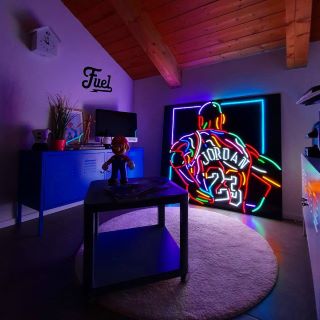This photograph showcases a dimly lit recreational or game room, filled with various eclectic items. Dominating the back wall is a vividly illuminated neon sign of Michael Jordan, presenting his back with the iconic "Jordan 23" jersey, outlined in a dazzling array of colors including white, blue, red, green, yellow, and purple. To the left, a television and a collection of knick-knacks are visible, contributing to the room’s playful ambiance. In the forefront, a dark-colored wheeled table stands on a circular cream-white carpet, proudly displaying a statuette of Super Mario. Adding charm to the space, a house-shaped clock and a "Fuel" banner adorn the wall, while a dark-colored desk, possibly blue, accompanies a computer and various small plants, enhancing the room's cozy and quirky vibe.